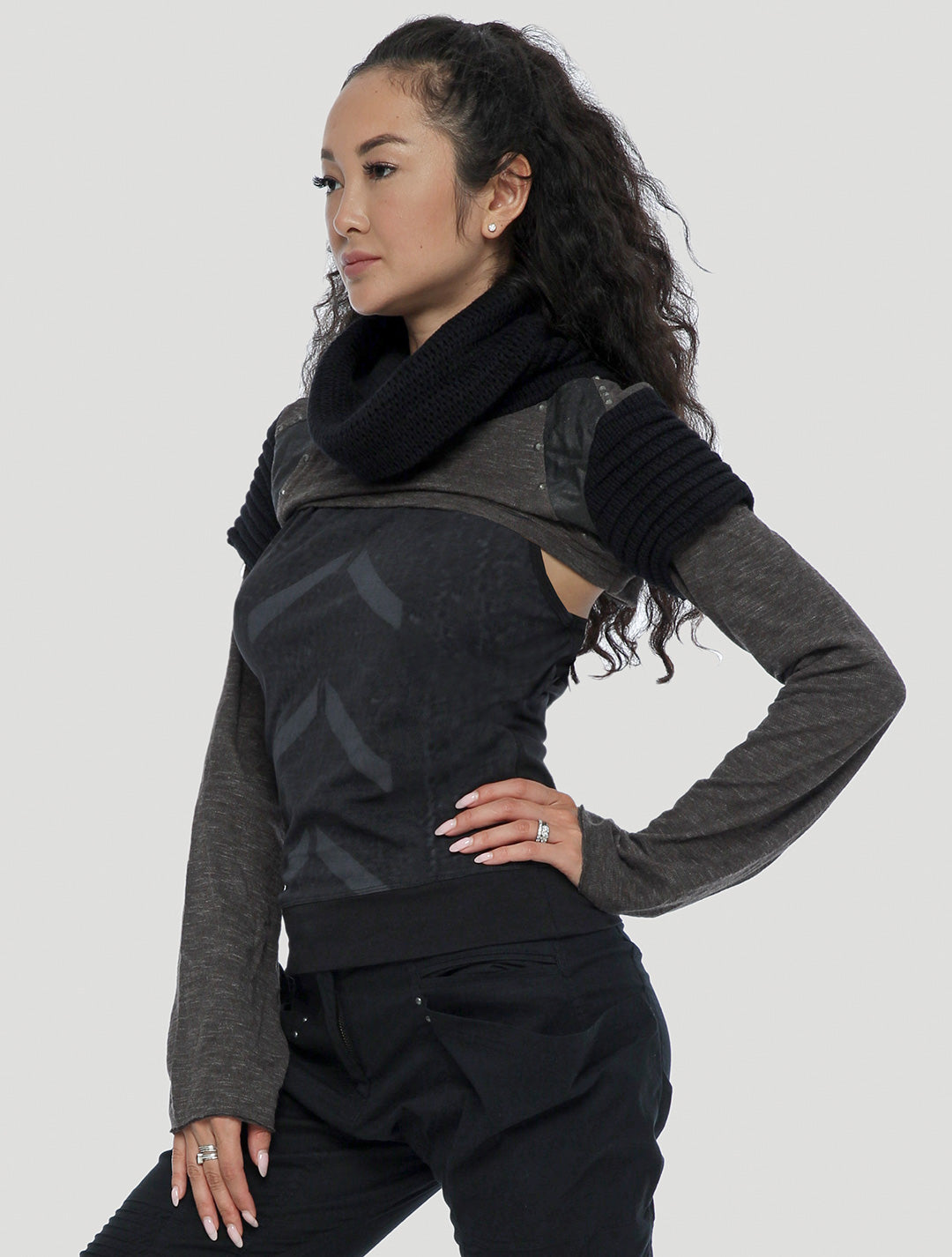In this fashion photograph, a young Asian model with long, wavy black hair cascading down to her mid-back is striking a posed stance. She gazes thoughtfully into the distance towards the left side of the frame. Her left hand, adorned with a sparkling diamond ring on her ring finger, rests confidently on her waist. Her left ear features a delicate diamond stud earring, while her right hand, with a ring on her middle finger, is placed elegantly on her inner thigh.

The model's ensemble is a layered combination of trendy pieces. She is clad in a dark gray long-sleeved shirt, over which she wears a black knit turtleneck, resembling an oversized scarf draping around her neck and shoulders. On top of this, she sports a cropped gray short-sleeved top that accentuates the upper segment of her outfit. Her black or very dark gray pants complete the sleek and sophisticated look. The careful positioning of her soft pink-painted nails adds a finishing touch to her poised and stylish appearance, making this photograph a quintessential example of contemporary fashion photography.